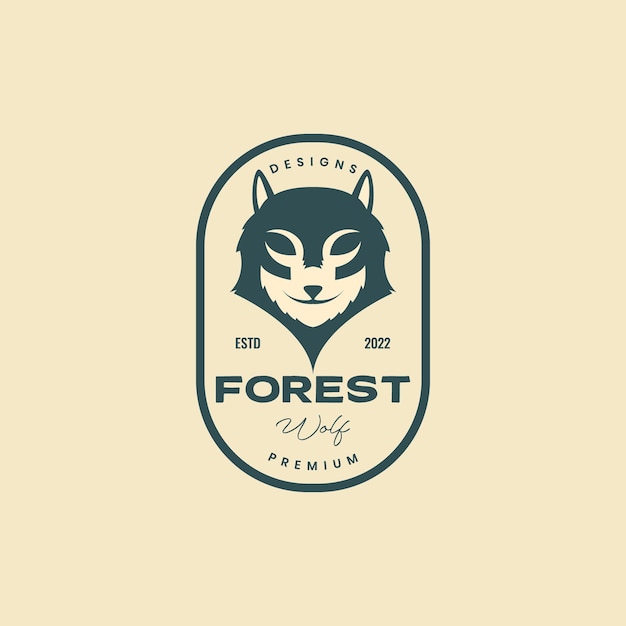The image features a logo with a dark green elongated oval border set against a cream-colored background. Within this border, the logo contains several elements arranged from top to bottom. At the top, the word "Designs" is written in small text, directly above a cartoony wolf head that is depicted in profile with ears pointed straight up and a smirking expression. The wolf's face is dark green, featuring an upside-down triangle nose and oval eyes, with cream-colored accents around the mouth and eyes that blend with the background. Below the wolf head, the text "ESTD 2022" is displayed, followed by the word "Forest" (noticeably missing an 'R'). Beneath this, the word "Wolf" is written in a script-like font, followed by the term "Premium" at the bottom. The logo's overall color scheme is restricted to dark green and cream, giving it a clean, minimalist appearance. The specific purpose of the logo—whether for clothing, food, or another category—is not indicated.